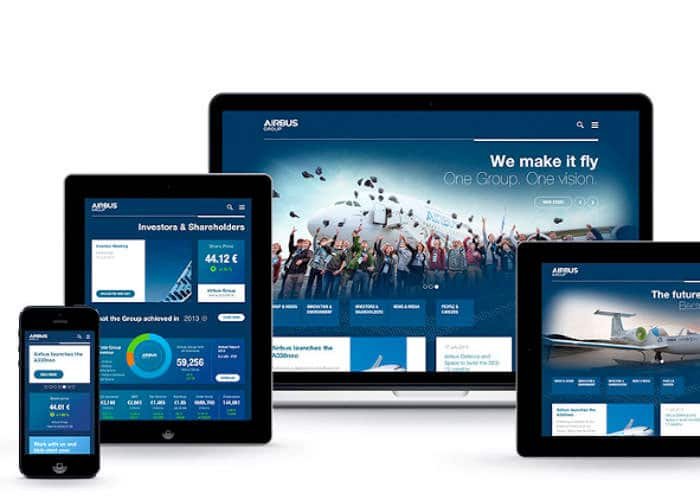The image prominently displays a multi-device advertisement for the Airbus Group website. Featured are several screens: a laptop, two tablets, and a smartphone, all showcasing the same foundational theme but with slight variations in content. Each device has a sleek silver frame with an inner black border, followed by a navy blue edge encircling the image itself. The top left corner of every screen displays the white "Airbus Group" logo. 

The main focus is on the central screen, which portrays a striking image of an Airbus airplane adorned with the company's name in white. Below the airplane, a group of people is seen joyfully tossing their hats into the air. The text overlay reads, "We make it fly - One Group, One Vision." 

The other screens present assorted content: one shows gathered data, another features an additional airplane image, and the composition finishes with the smartphone placed in the lower left. To its right is a tablet, with a laptop in the background and another tablet on the far right. The consistent color scheme and design elements create a cohesive visual experience across all devices.